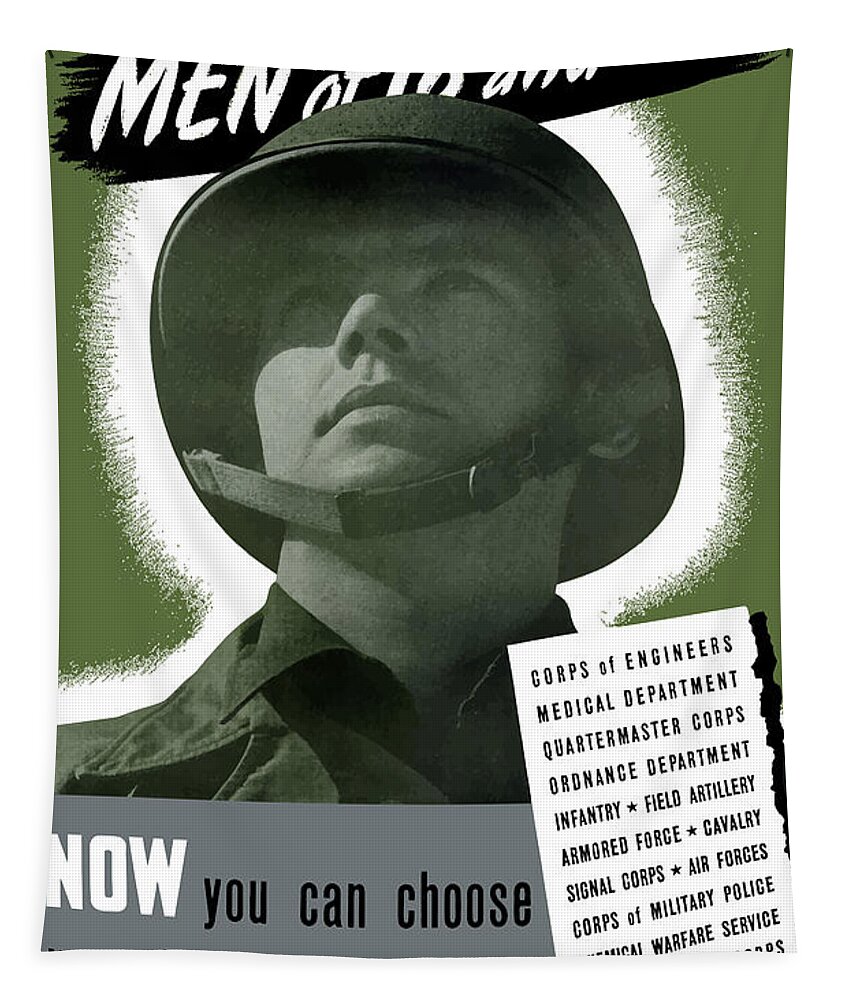The image is a vintage military recruitment poster featuring a prominently displayed soldier’s face, front and center. The soldier wears a classic army helmet with a leather chin strap, and his expression is one of resolute determination as he gazes slightly upwards to his left, toward the sky. He dons a military-style coat in dark green hues that blend seamlessly with the green-tinted background. A white, sunburst-like outline encircles his head, enhancing the heroic aura.

Above the soldier's head, a partially obscured black banner with white text reads "men of," with the remainder of the phrase cut off. Below this segment, a gray rectangle bears the phrase "now you can choose," in dual-color text: "now" in white and "you can choose" in black. Adjacent to this, in the lower right corner, a white background section lists the various military branches one can join, including the Corps of Engineers, Medical Department, Quartermaster Corps, Ordnance Department, Infantry, Field Artillery, Armored Force, Cavalry, Signal Corps, Air Forces, and Corps of Military Police. The entirety of the design evokes a sense of historical significance, reminiscent of World War II-era enlistment appeals.